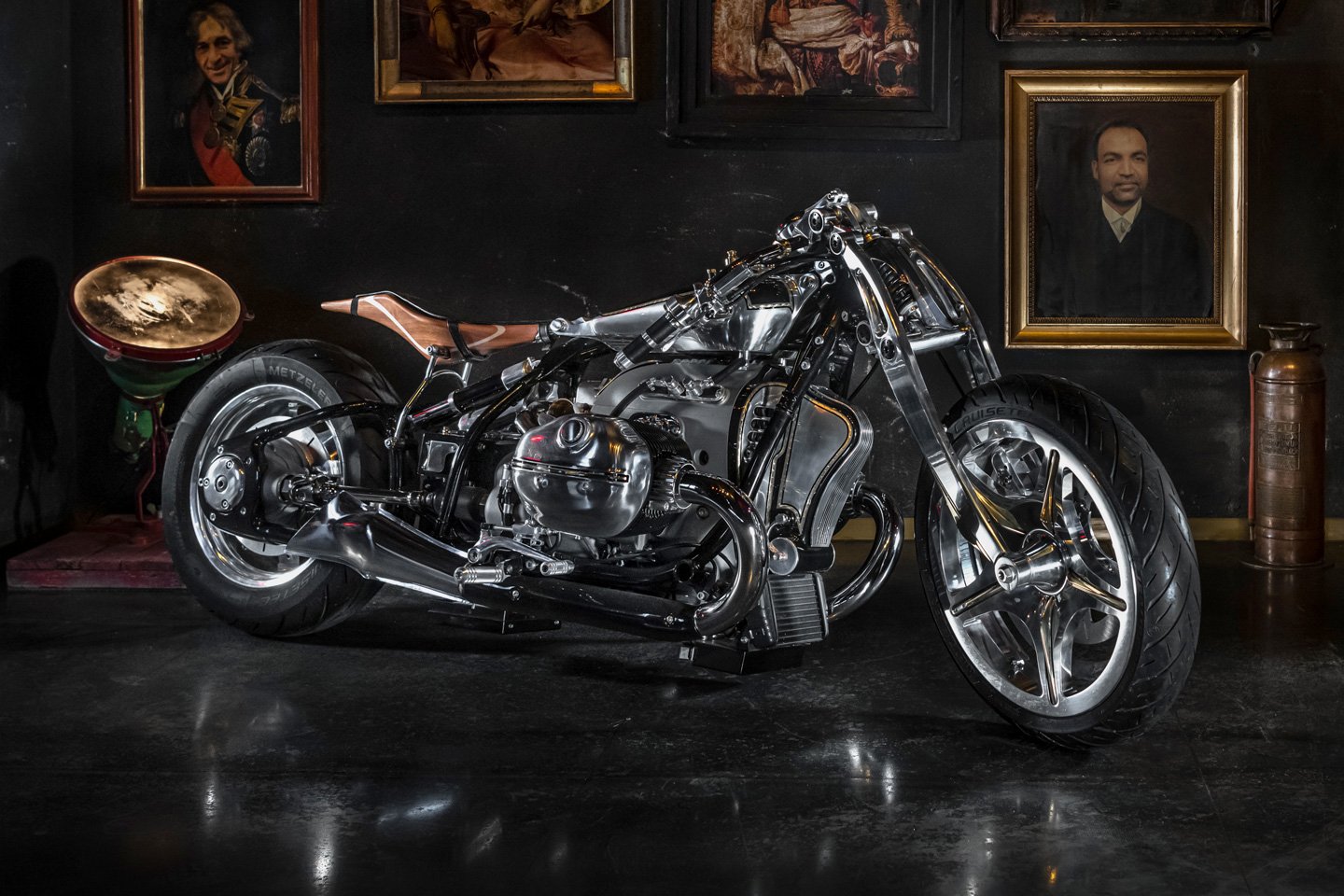The image captures a pristine motorcycle, prominently showcased within what appears to be a sophisticated showroom. The motorcycle features a sleek, shiny silver metallic body, possibly even platinum, accentuated with black-painted elements such as the exhaust, steel structures near the tail, and parts of the frame. The seat is a contrasting brown, resembling a bucket seat with visible springs below.

The motorcycle stands on a shiny, black reflective surface, meticulously polished to mirror the lights that are out of view. The backdrop features a black wall adorned with various portraits, the most notable being a man in a suit, framed in gold, located to the right of the motorcycle. Just to the bottom right corner of this prominent portrait, a bronze-colored fire extinguisher or a pressurized gas cylinder rests on the floor, adding to the room's eclectic charm.

Overall, the setting exudes an air of elegance and modernity, with clear, bright natural lighting enhancing the clarity of the image and highlighting the meticulous details of the motorcycle and its upscale environment.